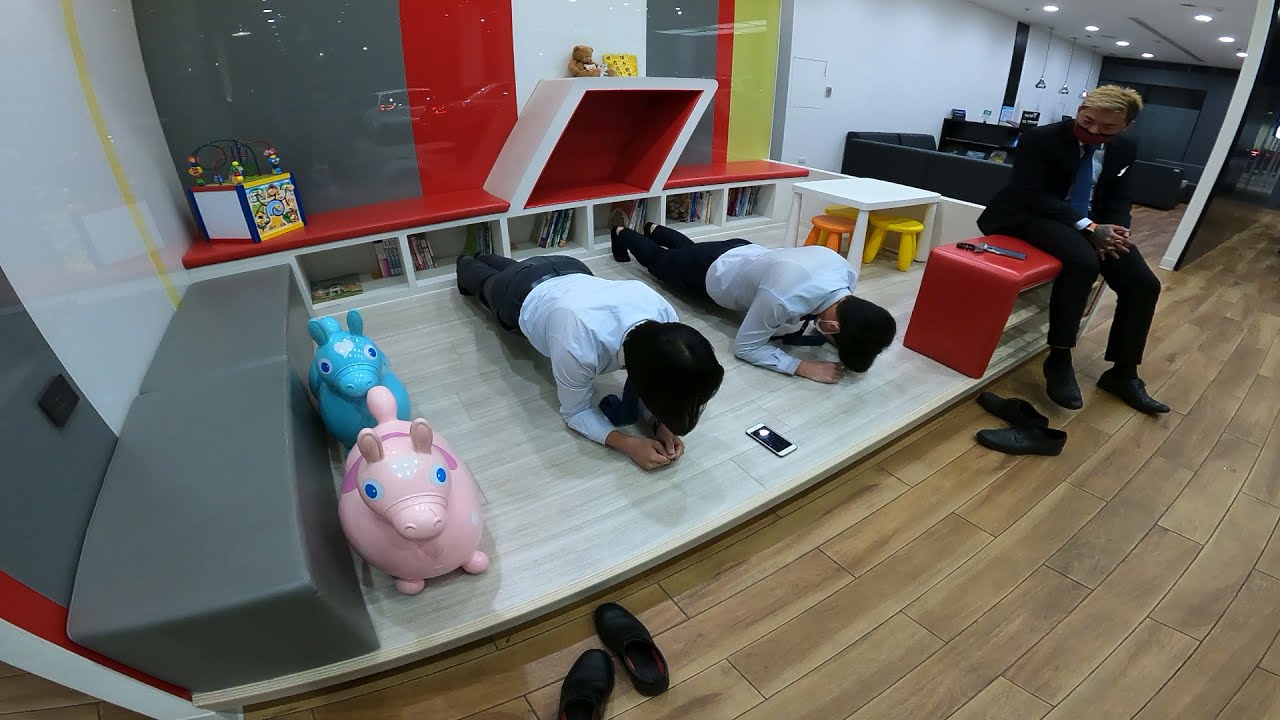In an indoor setting with white walls and hardwood floors, the image depicts a scene that could be set in an office or a kindergarten room. The main focus is on two individuals wearing light blue collared shirts and black dress pants, positioned on a small platform, appearing to perform planks or a similar exercise with their elbows and toes touching the ground. Beside them are two stuffed animals—a pink and a blue hippo—indicating a mix of professional and playful elements in the environment. Additionally, a third man dressed in a black suit with a white shirt and a blue tie, with blonde dyed hair, sits on a red bench, observing the two individuals. His shoes are on while the others have removed theirs, which are placed on the floor in front of the platform. The room is well-lit by ceiling spotlights and features some black couches and shelves with books. A designated children's area is visible, equipped with a white table, small yellow and orange chairs, and various toys, contributing to the playful atmosphere. A solitary cell phone rests on one of the surfaces, adding to the detailed portrayal of the setting.